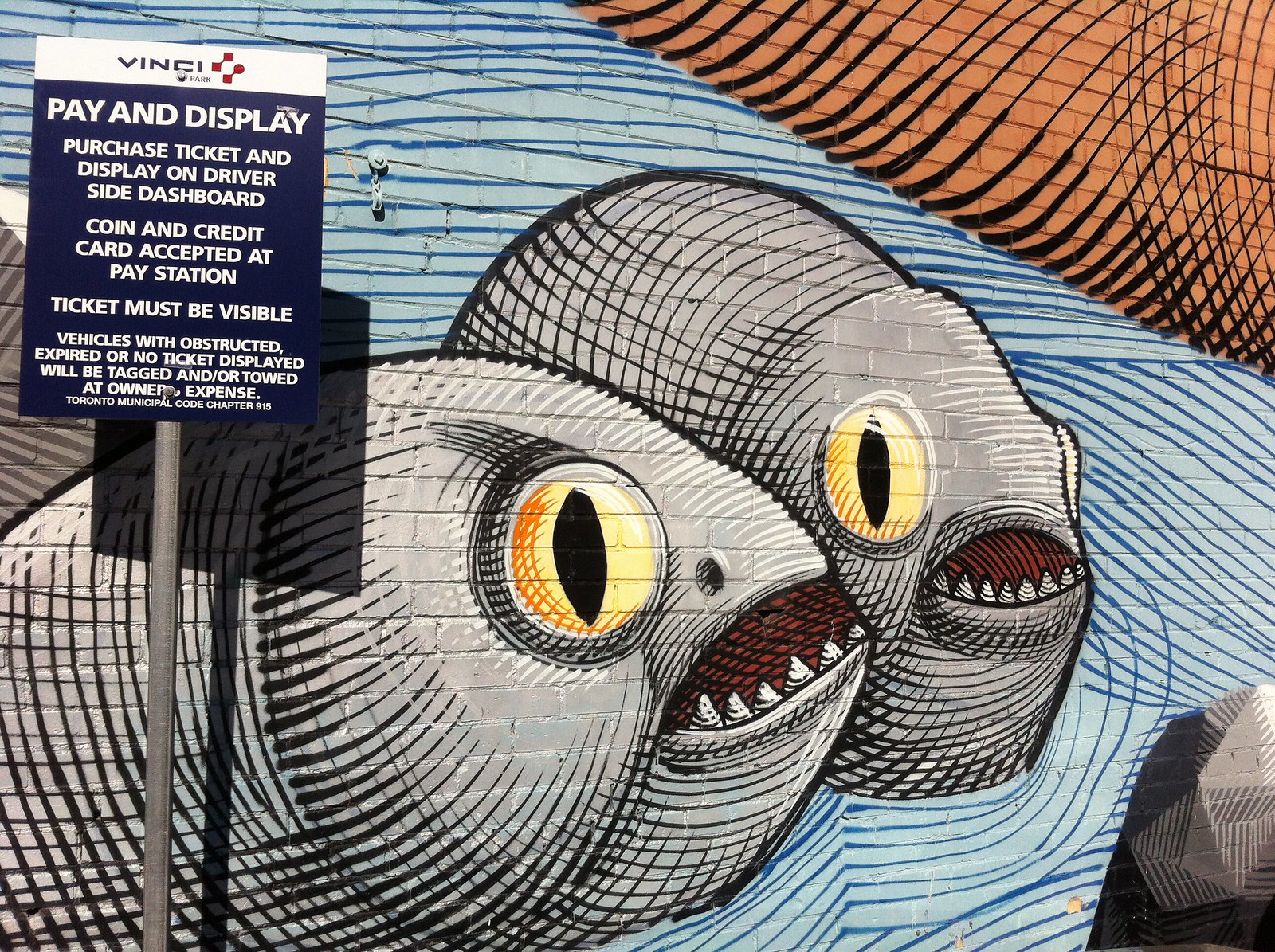The image showcases a detailed, painted mural on a brick wall, depicting two large, gray fish that resemble piranhas with their wide-open mouths revealing jagged teeth on their bottom jaws. They have haunting, big golden-yellow eyes with black irises, set against a vivid blue water background with light and dark blue lines. In the mural, the fish appear to be swimming near the brownish ground visible at the top left and right corners.

In front of this mural stands a parking sign affixed to a gray metal pole. The sign has a distinctive design with "Vinci" at the top, highlighted by a red cross on a white background. Below this, on a navy blue section, the sign instructs: "Pay and Display" along with, "Purchase ticket and display on driver's side dashboard." It also states, "Coin and credit card accepted at pay station. Ticket must be visible. Vehicles with obstructed, expired, or no ticket displayed will be tagged and/or towed at the owner's expense." At the bottom of the sign, in smaller white font, it reads "Toronto Municipal Code Chapter 915." The mural and the parking sign together suggest that the area is part of a pay-to-park zone.